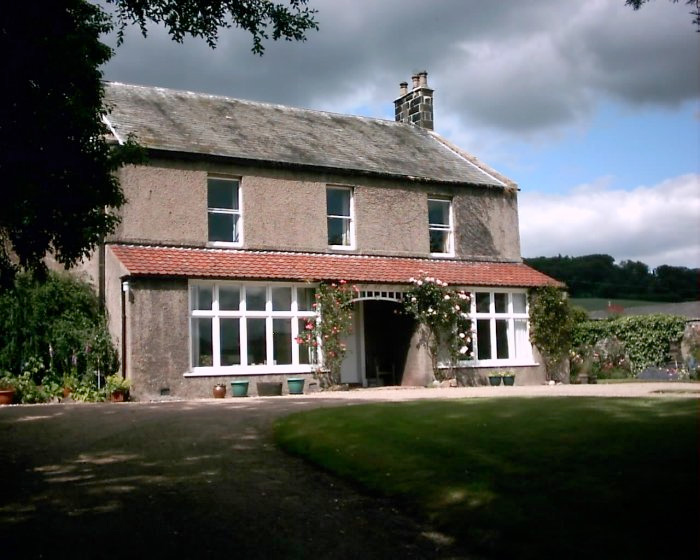The photograph captures a two-story building set in a countryside area, framed by a light blue sky with ominous dark grey clouds overhead, suggesting an outdoor daytime setting. The foreground prominently features a gravel path that loops around a small, flat green yard. The building, constructed of small grey bricks, boasts a lower front roof made from red tiles and an upper roof that is dark grey, mottled with white and various darker stains. The structure includes multiple windows with white frames on the top right. To the left, trees cast significant shade over the scene, hinting at an abundance of foliage nearby. The shot is taken from a distance, approximately 70 yards away, placing the building centrally within the image. The background includes a hint of rustic trees, adding further depth to the serene, countryside ambiance.